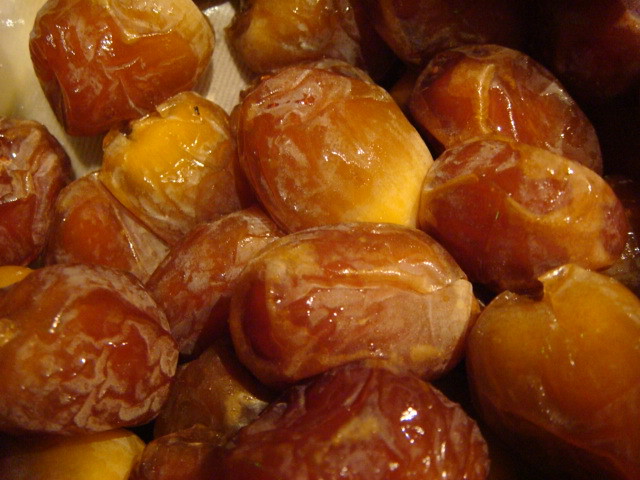The image depicts a close-up view of what appears to be a pile of small, egg-shaped fruits, possibly dates or a similar dried fruit. These fruits display a range of colors from orange at the top to yellow at the bottom, with some showing a golden-brown hue from cooking or baking. The skins are slightly wrinkled, indicating they've been dried, and they possess a glistening, sticky appearance that suggests either a glaze or inherent moisture. The fruits are nestled on an off-white, ribbed paper, and some of them extend into the darkness at the top right corner of the image, implying there may be more out of the frame. The ends of the fruits show signs of where stems might have been attached, or they are opened as if pits had been removed. Overall, the clustering of around 18-20 fruits fills the entire visual frame, highlighting their glossy and slightly hazy texture.